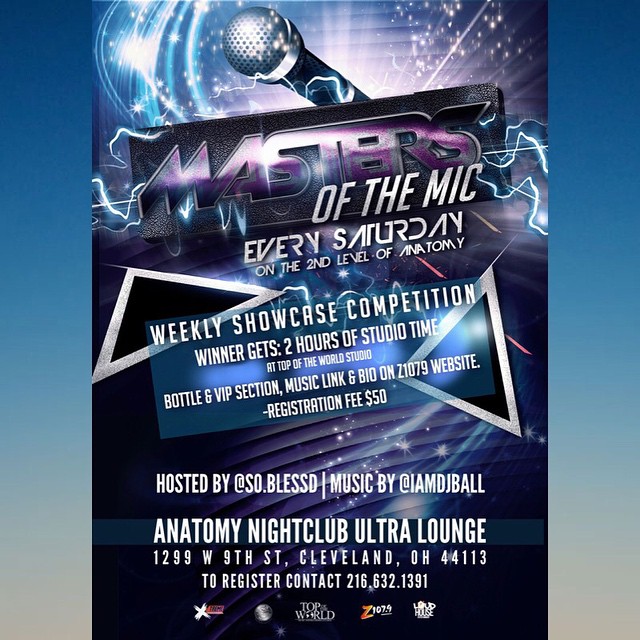The image is an advertisement poster for an event titled "Masters of the Mic," hosted every Saturday on the second level of the Anatomy Nightclub Ultra Lounge located at 1299 West 9th Street, Cleveland, Ohio, 44113. The top of the poster features an illustration of a microphone pointing to the top left, surrounded by electric sparks and shiny wave lines in blue and white. The event title, "Masters of the Mic," is displayed diagonally in large purple text with white lights illuminating the 'S' and varying brightness between the upper and lower halves of the letters. Below this, the caption "Every Saturday on the second level of Anatomy" is stated in bold white capital letters. There is a light blue transparent box that provides details about the event: "Weekly Showcase Competition. Winner gets two hours of studio time at Top of the World Studio, bottles, and VIP section. Music link and bio on Z 107.9 website. Registration fee $50." The event is hosted by @so.s0.bless with music by I AM DJ Ball. Contact information for registration is provided (216-632-1391). The bottom of the poster includes multiple sponsor logos.